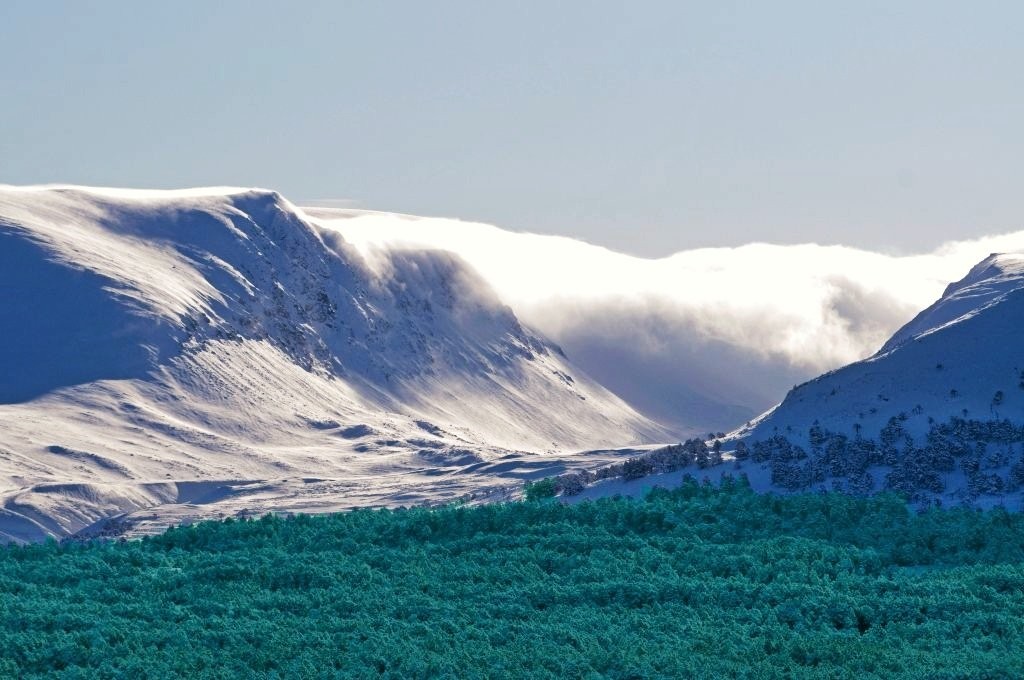This is a detailed photograph capturing a breathtaking mountain scene. The central focus is on a majestic mountain range featuring two prominent snow-covered peaks, one on the left and one on the right, with a valley nestled between them. The peaks are adorned with icy formations, and gray rocks are visible through the snow.

In the foreground, a dense array of green trees is clearly visible, indicating evergreen species, with some sections dusted in snow while others remain lush and untouched by it. As the trees descend the mountainsides towards the valley, the snow gives way to a verdant expanse, creating a striking contrast. 

The sky overhead is a soft blue, adding to the serene atmosphere, while a large white cloud or mist lingers in the valley, adding an element of mystery. This mist partially conceals the background, enhancing the depth of the image. Additionally, sunlight illuminates the side of one peak, suggesting that the sun is breaking through the clouds above.

Overall, this scene captures the serene beauty and contrasting elements of a snowy mountain landscape amidst a verdant forest, wrapped in a frame of a clear, slightly blue sky interspersed with mist.